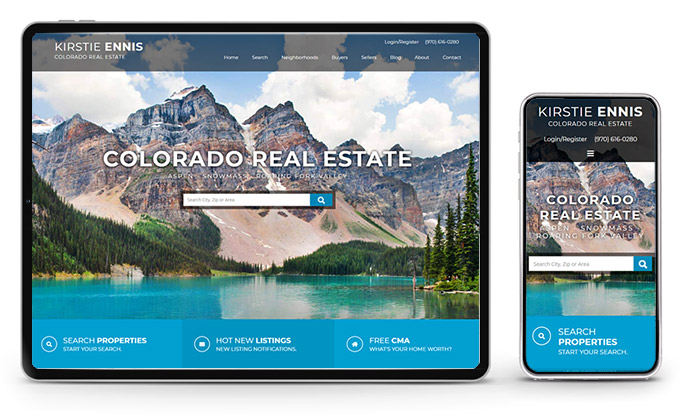The image on the left shows a laptop screen, while the image on the right captures a cell phone screen. Both screens display identical content. At the very top, there's a light gray banner, spanning from left to right, featuring "Christie Ennis Colorado Real Estate" in white text. Below this banner, the picturesque backdrop showcases a rugged and jagged set of mountains in various hues of gray, black, orange, and tan, with streaks of snow interspersed. At the base of these majestic mountains lies a dense forest of evergreen trees, leading into the foreground where a large blue lake glistens.

The gray banner at the top contains several menu options from the center to the right: Home, Search, Neighborhoods, Buyers, Sellers, Blog, About, and Contact. Central to the image, overlaying the mountains, are the words "Colorado Real Estate" in bold white text. Beneath this heading is a rectangular search box, predominantly white, with its right end highlighted in blue. The blue segment contains a magnifying glass icon in white, and the search box is inscribed with placeholder text: "Search city, state, zip, or area."

Spanning the bottom of the image are several clickable options in text: "Search Properties, Start Your Search," "Hot New Listings, New Listing Notifications," and "Free CMA, What’s Your Home Worth."